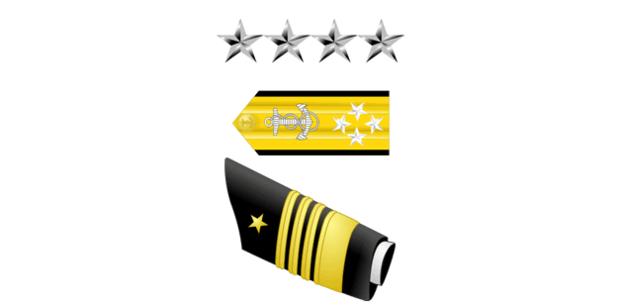This image showcases a series of military insignia against a white background, arranged in three distinct rows, each illustrating different decorative metal badges commonly used in military uniforms. The top row features four silver stars, glimmering with reflective highlights. The middle row displays a golden ribbon adorned with a black border on both the top and bottom edges. Centrally placed on this ribbon are four white stars encircling a white anchor symbol, with the background alternating between yellow and black stripes. The bottom row consists of a black badge with three horizontal yellow stripes and a prominent gold star, which along with the stripes, contrasts sharply against the black cloth material. The intricate designs provide insight into the detailed heraldry used for military identification and decoration.